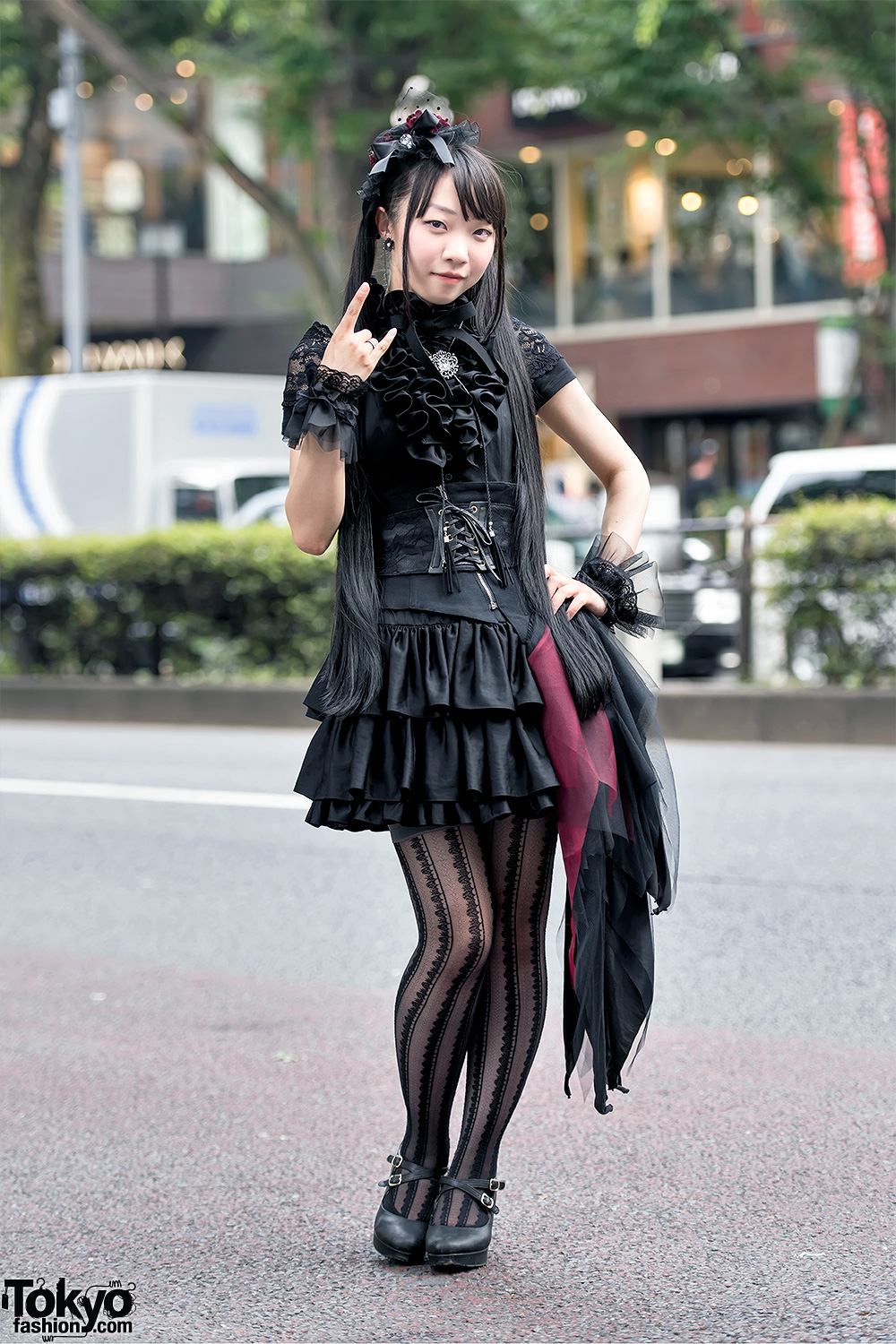This vertically aligned rectangular photograph captures a young Asian woman standing in the middle of a road. She has long, straight black hair with bangs and is adorned with a black bow. Her outfit is a short, ruffled black dress with sleeves that extend a little below her shoulders and down her biceps. She pairs this with striped black stockings and black sandals. Both her wrists are adorned with black lacy bracelets. The woman strikes a confident pose, with one hand on her hip and the other raised in a gesture, with her forefinger and pinky up while the other fingers are down. 

In the lower left corner of the image, the text "tokyofashion.com" is visible in black font. The background, though blurry, indicates an urban setting with a two-story building featuring upper-level windows with light streaming through. Several trucks are either parked or moving on the far side of the road, which is bordered by a row of bushes separating the lanes. The scene appears to be captured during the daytime in a business district.